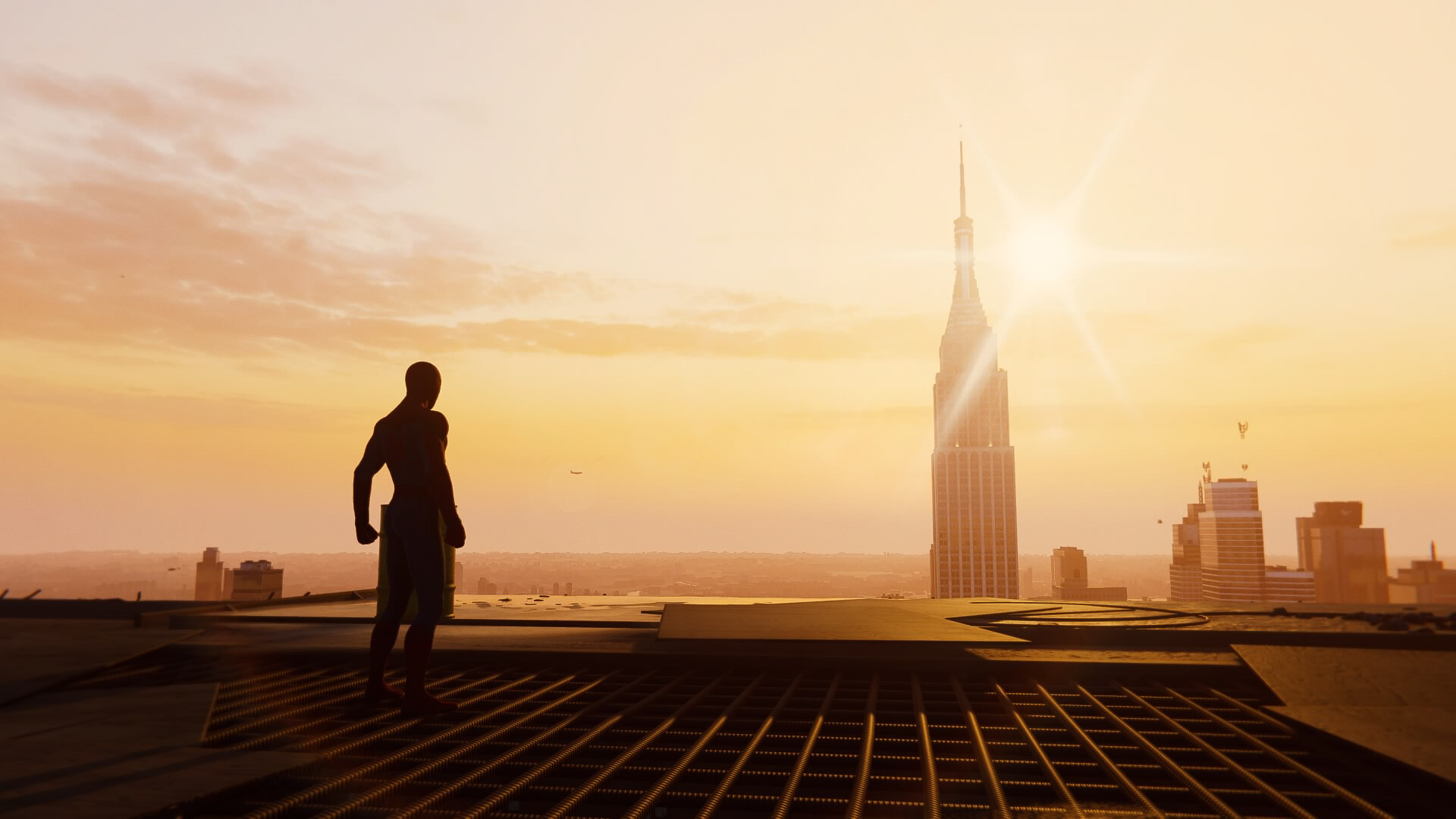This captivating digital artwork captures a powerful moment as a muscular, bald man stands on a rooftop, facing towards the sunrise. The image, slightly wider than it is tall, is bathed in a peachy-orange hue, giving it a warm and ethereal glow. The scene is dominated by a sky filled with both white and yellow clouds, through which the bright sun shines intensely from the top right corner, casting its luminescent light across the image.

The man is positioned roughly 30% from the left edge and about 10% up from the bottom, standing with his arms at his sides and fists clenched. His defined shoulders and biceps are clearly visible, emphasizing his strong build. He's either wearing shorts or a towel around his waist. The ground he's standing on appears to be an iron crisscross structure, typical of a commercial building's rooftop.

In the background, towering buildings rise towards the sky, with one particularly tall skyscraper—reminiscent of the Empire State Building—standing at about 60% from the left. These buildings are surrounded by shorter structures, completing the urban skyline that juxtaposes the serene and majestic sunrise. The combination of these elements creates a harmonious blend of human strength and natural beauty, captured in a moment of quiet reverence towards the rising sun.